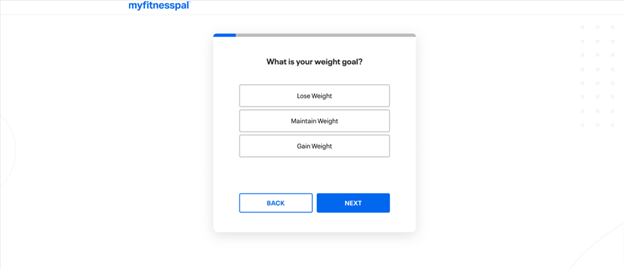The page predominantly features a stark, minimalistic design. In the upper left corner, a bold gray line runs vertically and horizontally, intersecting at 90 degrees. To the right of this intersection, the page remains largely open, with three vertical rows of dots subtly arranged in a very faint gray, tallying up to 21 dots.

On the left side, prominently displayed in blue, bold-face letters, is the text "MyFitnessPal." Below this header, a box with a shadow effect appears. In the upper left corner of this box, a blue line is visible, transitioning into a gray line extending horizontally to the right. Inside the box, bold-face type asks the question "What is your weight goal?"

Three rectangular boxes outlined in gray and filled with white are listed below the question:
1. The first box reads "Lose Weight."
2. The second box reads "Maintain Weight."
3. The third box reads "Gain Weight."

At the bottom of the page are two navigation buttons: "Back" on the left and "Next" on the right.